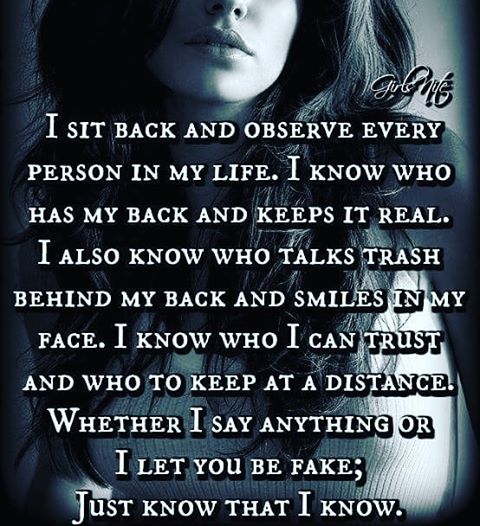The image is a poster or a frame from a PowerPoint presentation featuring an impactful photograph of a young woman. The photograph captures only the lower part of her face, focusing on her pouty lips, and extends to her upper torso. She appears to be wearing a white sweater, and her long, flowing dark hair is visible. The background, a blue and white photograph, provides a striking contrast to the message overlaid on it.

In bold, uppercase white font, the text on the image reads: "I sit back and observe every person in my life. I know who has my back and keeps it real. I also know who talks trash behind my back and smiles in my face. I know who I can trust and who to keep at a distance. Whether I say anything or I let you be fake, just know that I know." This powerful sentiment addresses themes of trust, observation, and authenticity, serving as a motivational and cautionary statement. 

Additionally, in the upper right-hand corner, "Girl's Night" is inscribed in a cursive font, suggesting a casual or intimate social context possibly targeted at young women who resonate with the message. The overall visual communicates a strong emotional undercurrent and serves as an assertive expression that might be shared on social media to convey awareness and self-assurance.